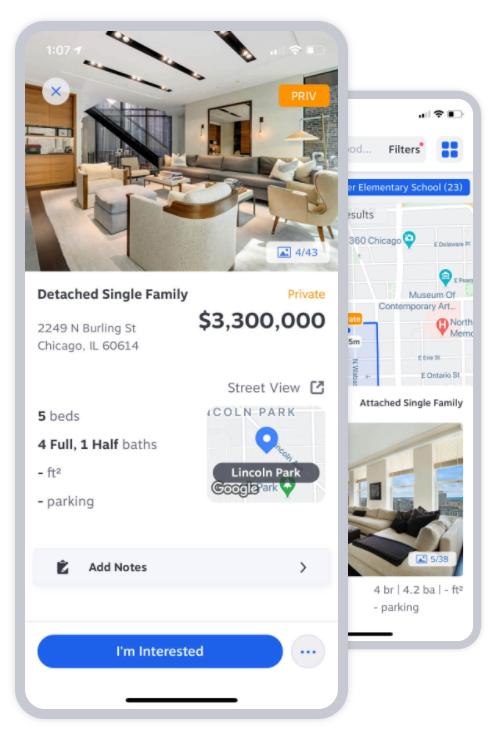**Image Description:**

This image, displayed on a cell phone screen, showcases a real estate listing for a house. The cell phone's status bar indicates a half-charged battery, a strong signal connection, and the time as 1:07. 

In the photograph, the focal point is the living room of the house, featuring a modern black staircase and cabinetry in the background. An orange box labeled "PRIV" appears prominently on the screen.

Beneath the photo, the property is detailed as a detached single-family home priced at $3,300,000. The listing includes the address located in Chicago and highlights the property amenities: five bedrooms, four full bathrooms, one half bathroom, and available parking. The orange box with "PRIV" is mirrored in a yellowy-orange color underneath the description.

A map section on the screen pinpoints the location in Lincoln Park with a blue marker featuring a white dot in the center.

At the bottom of the phone screen, there is a gray area with a "Add Notes" option and an arrow pointing to the right. Adjacent to this, an oblong blue "I'm interested" button is displayed alongside a smaller gray circle containing three dots, indicative of additional options.